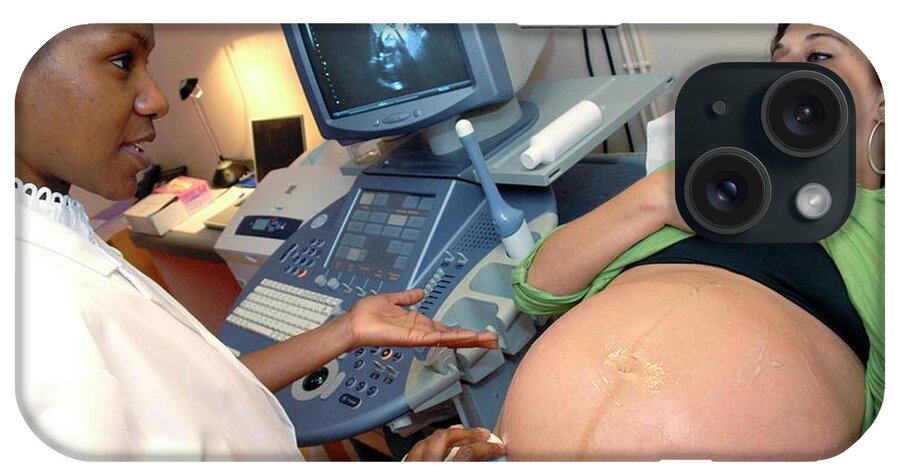This detailed iPhone case design features a vivid superimposed image of a pregnant woman during an ultrasound procedure. The scene captures an African-American doctor wearing a white coat, operating an ultrasound machine while the patient, dressed in a green shirt pulled up over her sports bra, lies on a bed. The doctor's attention is focused on a sophisticated machine adorned with numerous buttons and a keyboard, displaying the baby's sonogram on the monitor. The woman's eyes and hoop earrings are visible, although her face is partly obscured by the iPhone's camera module fitting positioned in the top left of the case. The entire photo, framed within the distinctive rounded rectangle of an iPhone 15, illustrates a heartwarming moment between the doctor and the expectant mother, making this phone protector uniquely personal and touching.